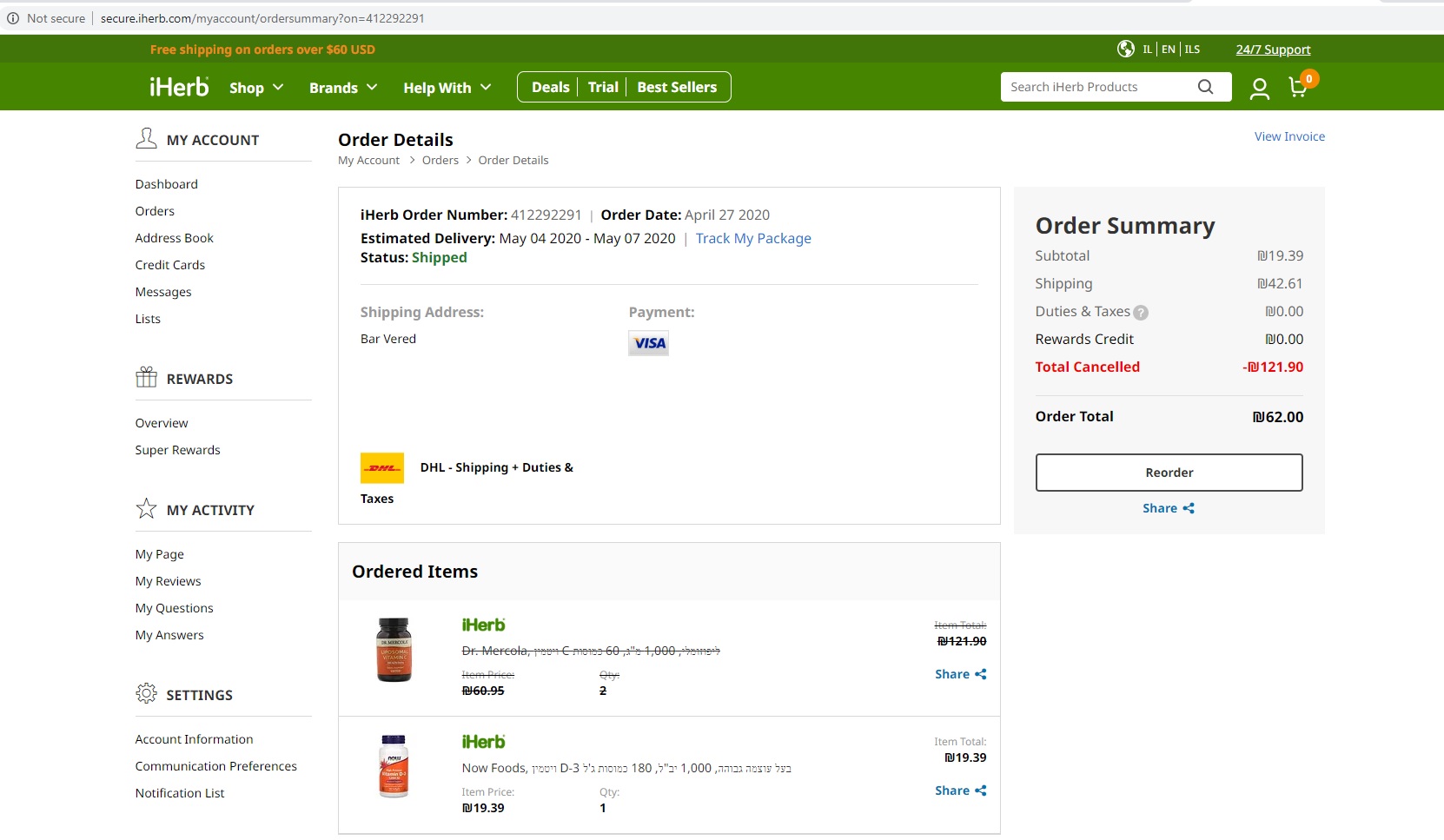This screenshot captures a webpage from the iHerb website. The top section features a dark green navigation bar that transitions into a lighter shade of green at the bottom. The website's logo, "iHerb," is displayed on the top left, with a lowercase 'i' followed by an uppercase 'H' and other lowercase letters in white text. Adjacent to the logo are navigation headers including "Shop," "Brands," "Help With," "Deals," "Trial," and "Bestsellers."

On the top right, there's a search bar and an option to switch the website's language, which is presumably set to English. Just above these options, "24-7 Support" is indicated. The screenshot also shows an icon indicating the user has six items in their cart.

The lower section of the screenshot reveals a confirmation page, detailing the items in the cart and the total amount paid. The items listed are pill bottles from Dr. Mercola and Now Foods, showcasing typical iHerb products. The total amount paid is shown as $6.62.